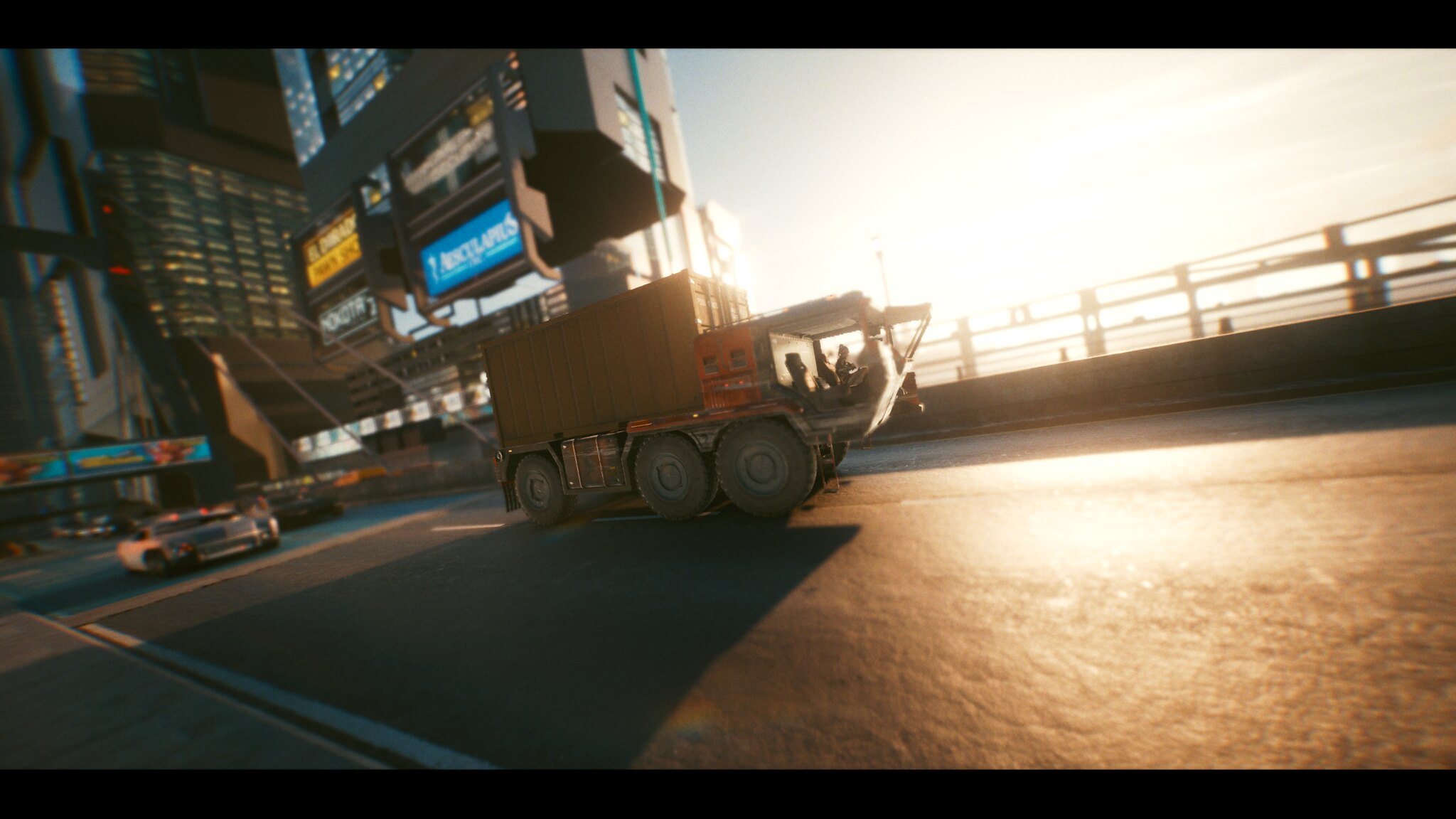In this color photograph, which gives off a cinematic vibe reminiscent of a video game screenshot, we see a bustling city street during dusk or possibly dawn, with the sun low on the horizon, casting a warm, orange glow over the scene. The main focus is on a large red truck with enormous tires and a copper-colored canister or container typically seen on freight tankers. The truck, somewhat translucent with glass sections, is driving towards the right side of the frame and is just about to transition onto a bridge, indicated by the change in the road color from lighter to darker black asphalt marked with white dashes.

Behind the truck, there are several vehicles, including a police cruiser and what appears to be a silver sports car. Additionally, on the left-hand side of the image, behind the truck, a city bus with a brightly lit turquoise sign on its top front can be seen. The photograph captures a part of an urban landscape dominated by towering skyscrapers, with one prominently featuring numerous small lighted signs, though the details of the signs are unreadable due to the distance. The perspective hints that the photographer was standing on the sidewalk, capturing the gleaming streets and the reflective surfaces of the vehicles under the tranquil yet vivid lighting of the setting or rising sun.